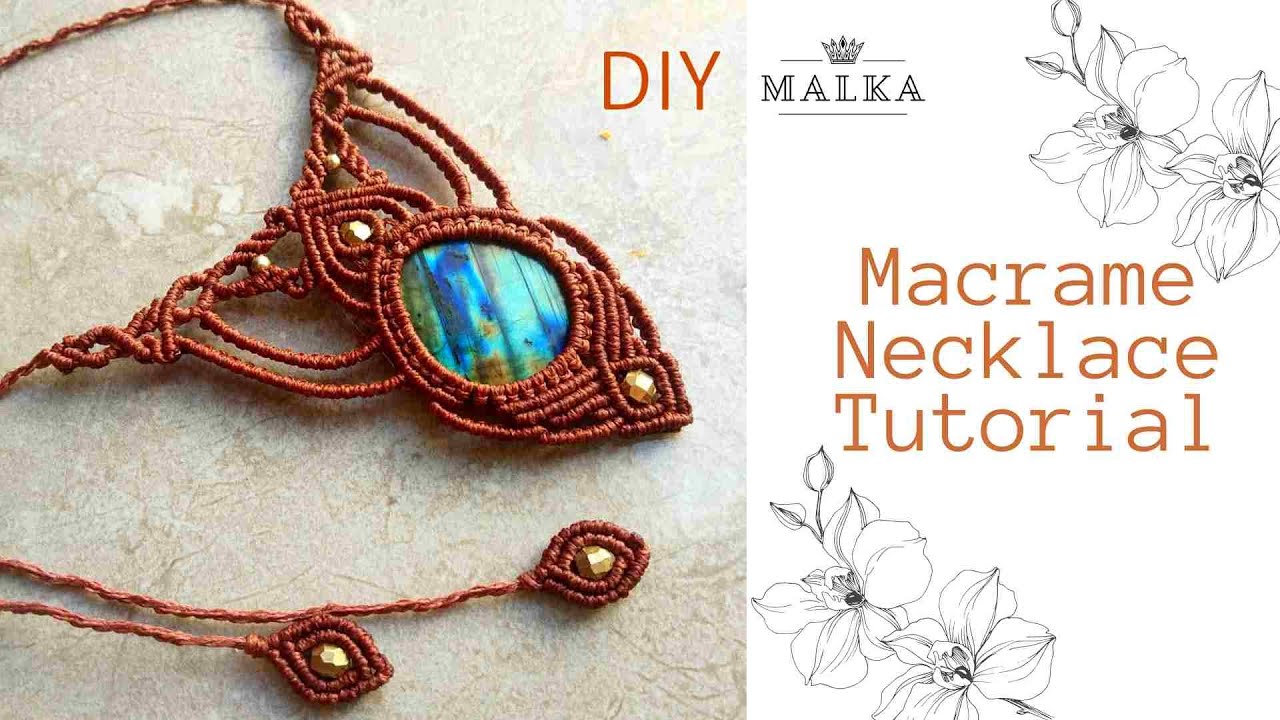The image shows a detailed macrame necklace tutorial advertisement. On the left, a photograph of a beautifully crafted, reddish-brown macrame necklace made of brown thread is set against a gray surface. The necklace features an eye-catching bluish crystal in the center. At its bottom, there are two tassels, each ending in a teardrop shape adorned with shiny golden beads. The necklace also incorporates intricate color patterns in shades of green, blue, and brown.

On the right, a drawing accompanies the photograph, highlighting key elements of the tutorial. In the top right corner of the drawing, decorative flower patterns can be seen, echoing similar motifs in the bottom left corner. The text "DIY Malka" appears at the top, with "Macrame Necklace Tutorial" prominently displayed in the middle. A distinctive crown logo with the word "Malka" is also positioned in the top left corner, adding a touch of branding to this high-quality, self-made necklace advertisement, encouraging viewers to sign up for the class.